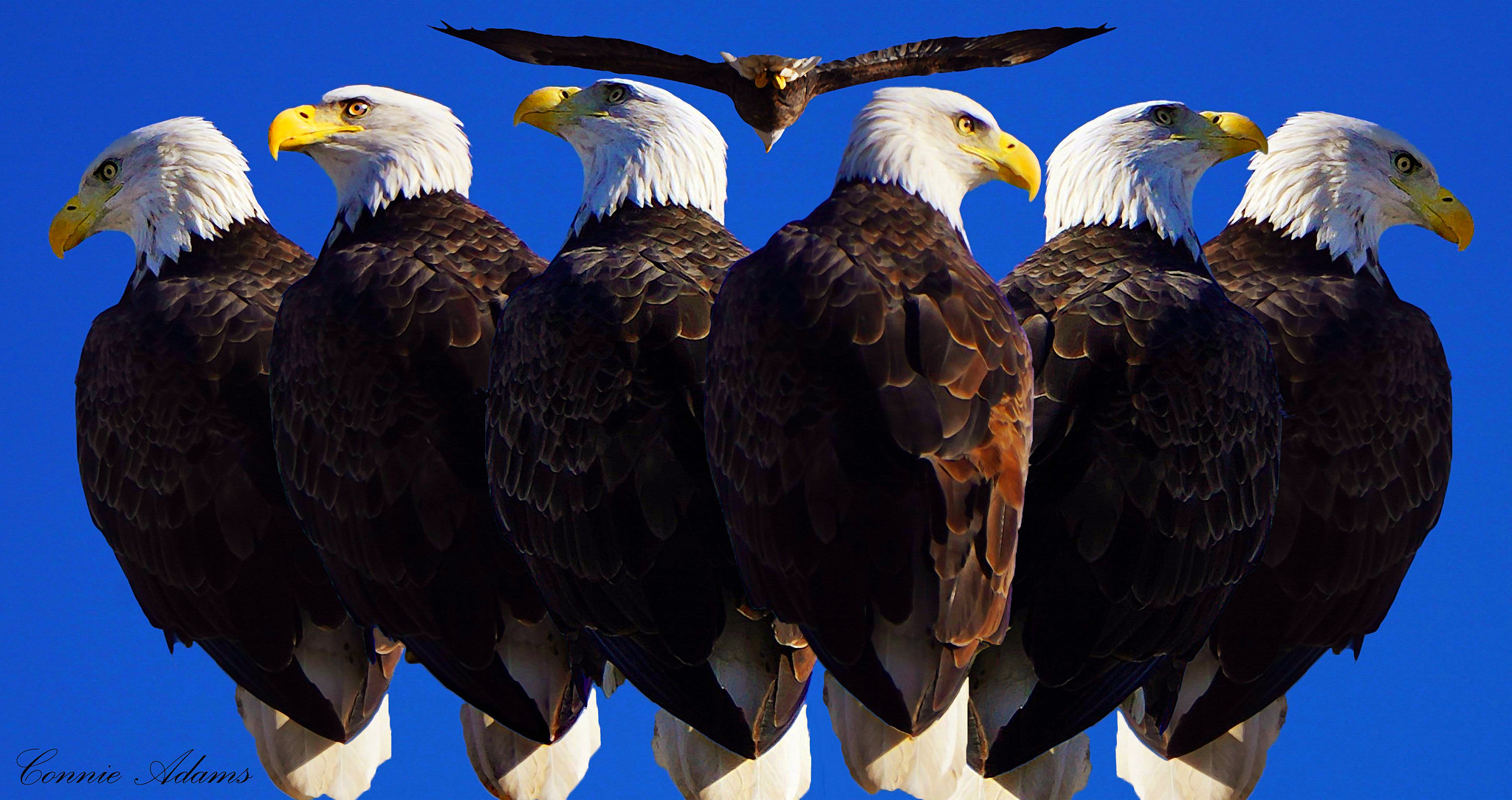The image showcases a striking composition by Connie Adams, prominently featuring six bald eagles and a hawk against a deep blue background. Signed in a black hand signature font on the bottom left, the image possibly combines photographs or computer-generated graphics to present an almost 360-degree view of the eagles. These majestic birds possess white head feathers, yellow beaks, brown bodies, and white tail feathers. The eagles are arranged in two symmetrical groups: on the right, three eagles profile to the right, and on the left, three eagles profile to the left. The variations in their head positions and angles offer a dynamic and detailed portrayal. At the top center of the composition, a hawk with black, flared-out wings and a white underside flies with a piercing gaze, adding a sense of motion and contrast to the static poses of the eagles below.